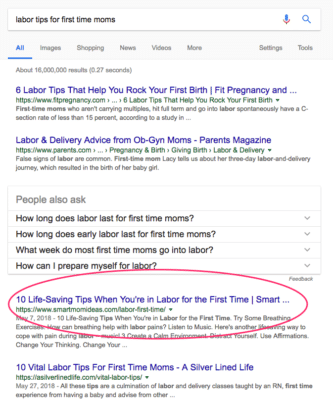The image displays a screenshot of Google search results, with the search query "labor tips for first-time moms" entered in the search bar at the top. Below the search bar are various options like "All," "Images," "Shopping," "News," "Videos," "More," "Settings," and "Tools," with the "All" tab selected. The search yielded approximately 16 million results in 0.27 seconds. 

Highlighted in the screenshot are several notable results. The first result is from FitPregnancy.com, titled "Six Labor Tips to Help You Rock Your First Birth," which emphasizes that first-time moms who are not carrying multiples, reach full-term, and go into labor spontaneously have a C-section rate of less than 15%, according to a study.

Additionally, there are "People Also Ask" questions with expandable drop-down options. A particular link is circled in red, indicating it was edited using a photo editing tool. This link is titled "10 Life-Saving Tips When You're in Labor for the First Time," from the website SmartMamas.com (smartmamas.com/labor-first-time/), dated May 17, 2018. The circled content suggests trying breathing exercises and explores the question, "How can breathing help with labor?"

Overall, the image provides a detailed snapshot of search results, focusing on essential labor tips and resources for first-time mothers.